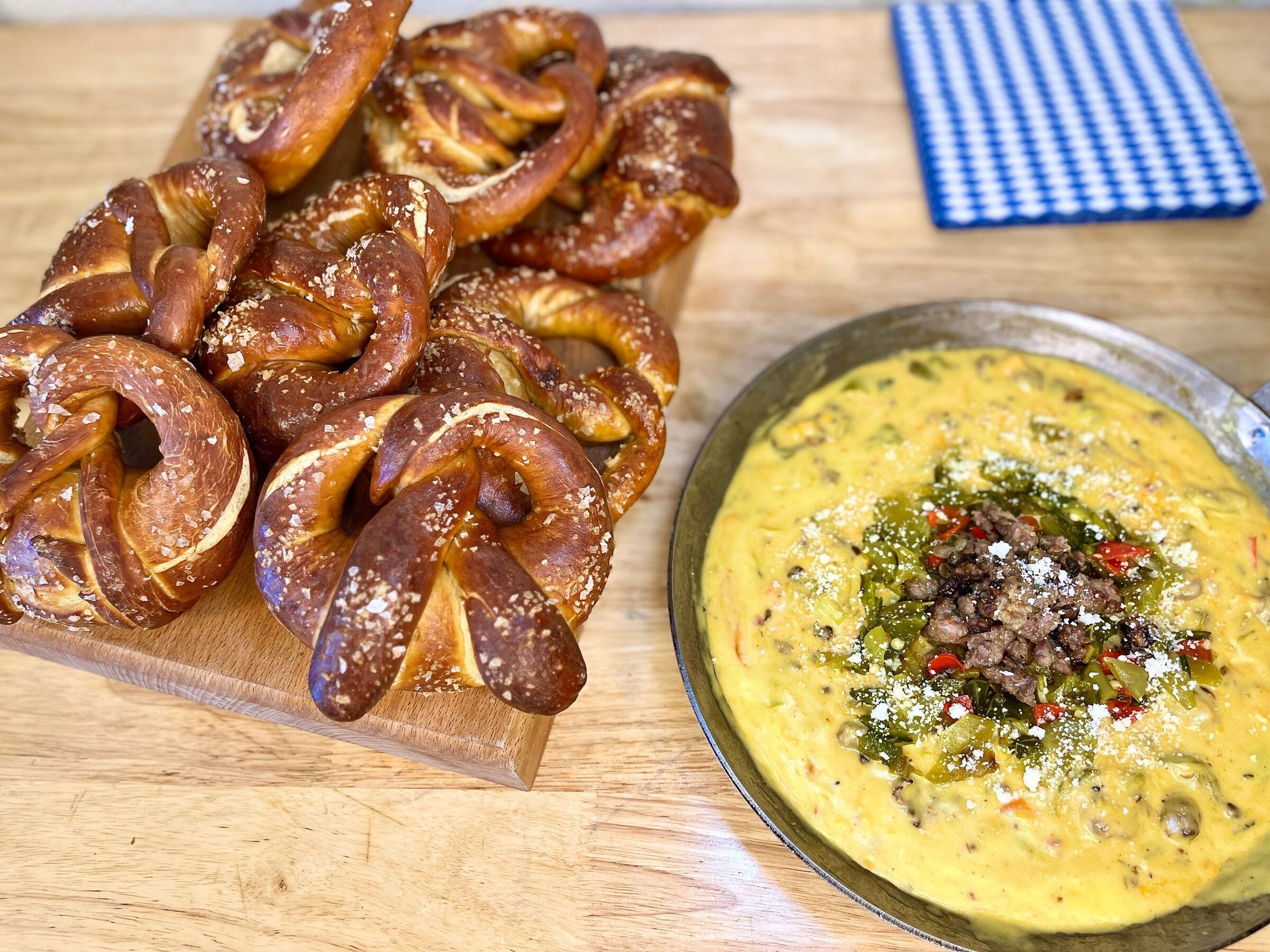The image depicts a wooden countertop with an arrangement of homemade pretzels and a dipping sauce. On the left side of the picture, there's a wooden cutting board stacked with about eight to nine beautifully browned pretzels, each generously sprinkled with coarse salt. In the bottom right corner, there's a shallow metal pan filled with what appears to be a rich, yellow dipping sauce, likely beer cheese or another type of cheesy dip. This sauce is seasoned with various herbs and spices, adding splashes of red, white, and green to its surface. A blue and white cloth napkin lies in the upper right corner of the image. The overall scene is set on light wood polished planks, with the objects arranged neatly for an appetizing display. The picture was taken from above, highlighting the contrasting colors of yellow, dark green, brown, light blue, white, tan, and dark brown, capturing a cozy indoor ambiance.